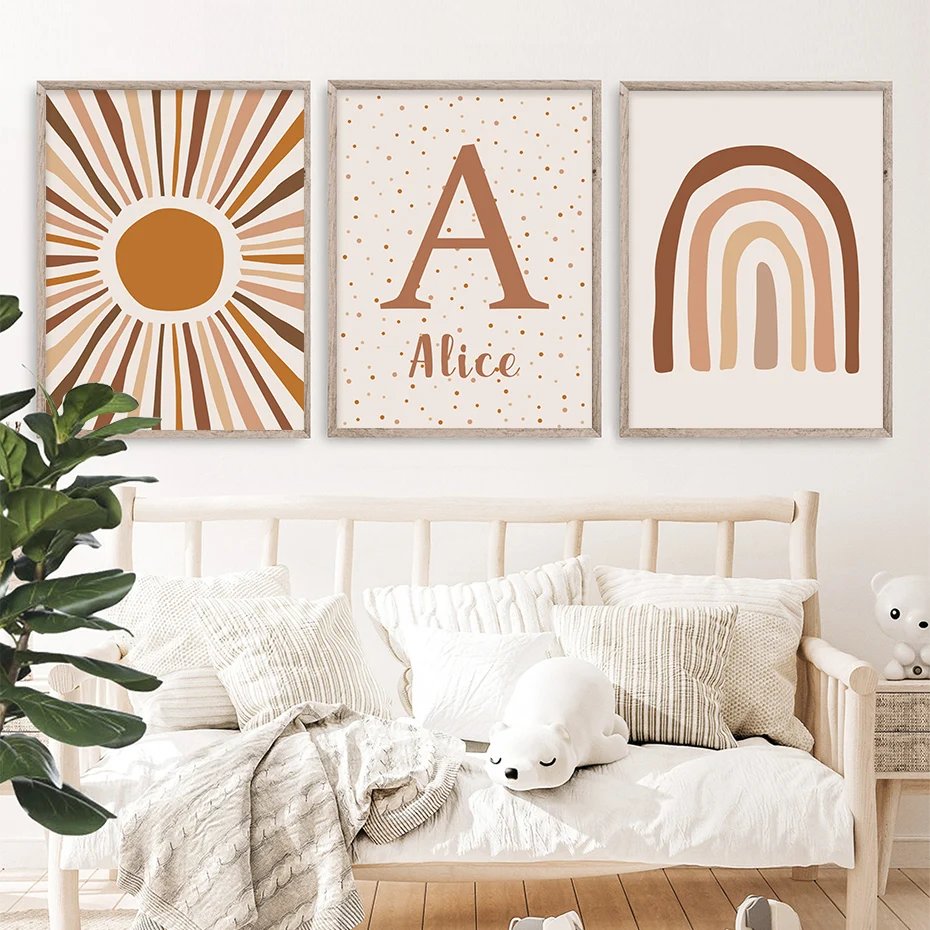This indoor photograph showcases a modernistic and simplistic sitting area, characterized by a white wall and hardwood floors. Central to the image is a wooden daybed or futon with a series of large, plush pillows in shades of white, beige, and tan. Draped over it is a soft throw blanket and, nestled among the pillows, is a polar bear stuffed animal. Adjacent to the daybed on the right is a rattan-style end table featuring a whimsical white anime-style bear figurine. A tall green plant with large rubber-like leaves peeks into the frame from the left, adding a touch of natural vibrancy to the room.

Above the daybed, three equally sized framed artworks are displayed, matching the color scheme of cream, tan, and dark brown. The leftmost artwork depicts a starburst design with beams radiating outward in various shades of brown. The central piece is a white background adorned with brown polka dots, prominently featuring a capital letter 'A' with the name 'Alice' beneath it. The rightmost image features a series of descending crescents or upside-down U shapes in transitioning shades of brown, creating a layered, rainbow-like effect. 

This cohesive design, with its blend of neutral tones and both organic and whimsical elements, suggests an aesthetically pleasing, serene living space that might be featured in a home interior decoration catalog.